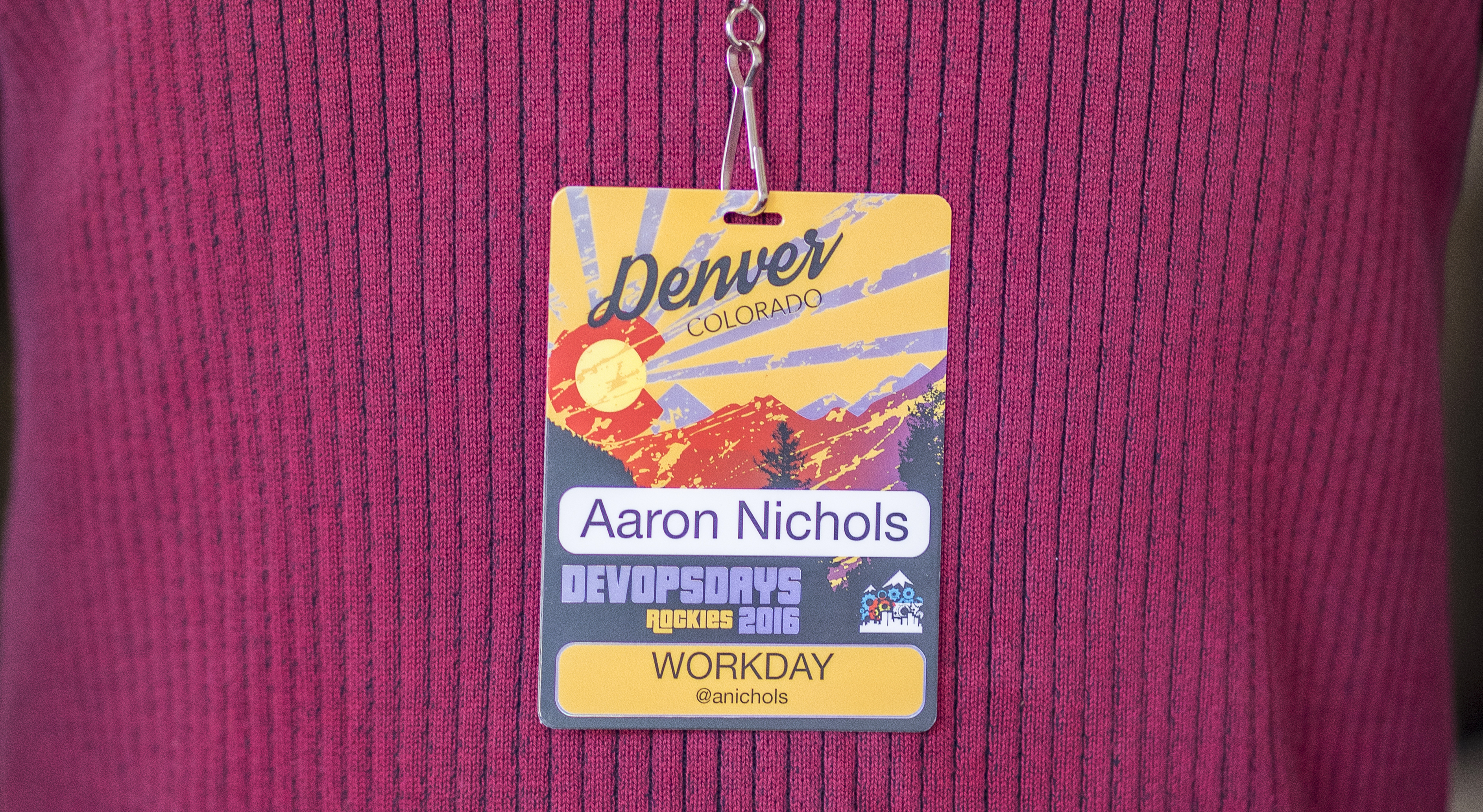The image showcases a badge from a convention, prominently featuring the name "Aaron Nichols" and the event "DevOps Days Rockies 2016" in Denver, Colorado. The badge, clipped to a lanyard with a noticeable metal clip, includes graphic design elements such as a sunset with rays extending over the Rocky Mountains, incorporating elements of the Colorado flag. Additionally, there is text indicating "@ANichols" as a social media handle and "Workday" near the bottom. The badge is worn by a person dressed in a distinctive sweater, which is primarily pink with sections of black or dark purple lines.